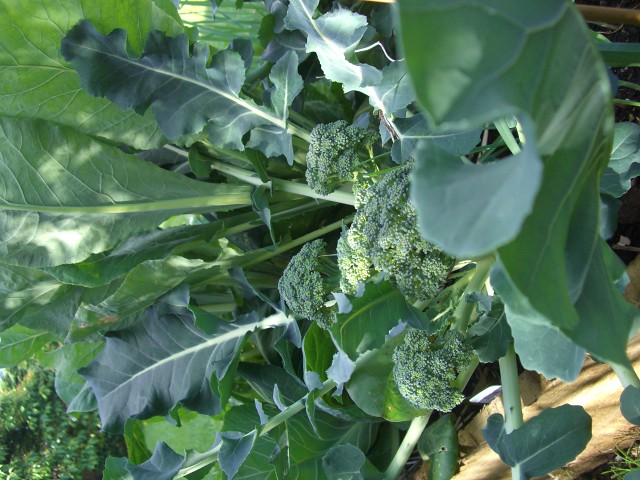The image shows a vibrant vegetable garden illuminated by patches of sunlight. On the right-hand side, there are long, skinny green leaves resembling loose-leaf lettuce. The darker green, textured leaves with a slightly curled pattern occupy the central portion of the image, where several heads of broccoli are prominently growing. These broccoli plants have substantial, billowy leaves that can span over 12 inches, shading parts of the garden and possibly preventing weed growth. On the left side, additional wide-stemmed green plants are visible, alongside an unidentified large leafed plant. In the lower left corner, there's a hint of something brown, potentially a wicker basket. Small green buds and grasses can be seen scattered throughout, adding to the garden’s lush composition.